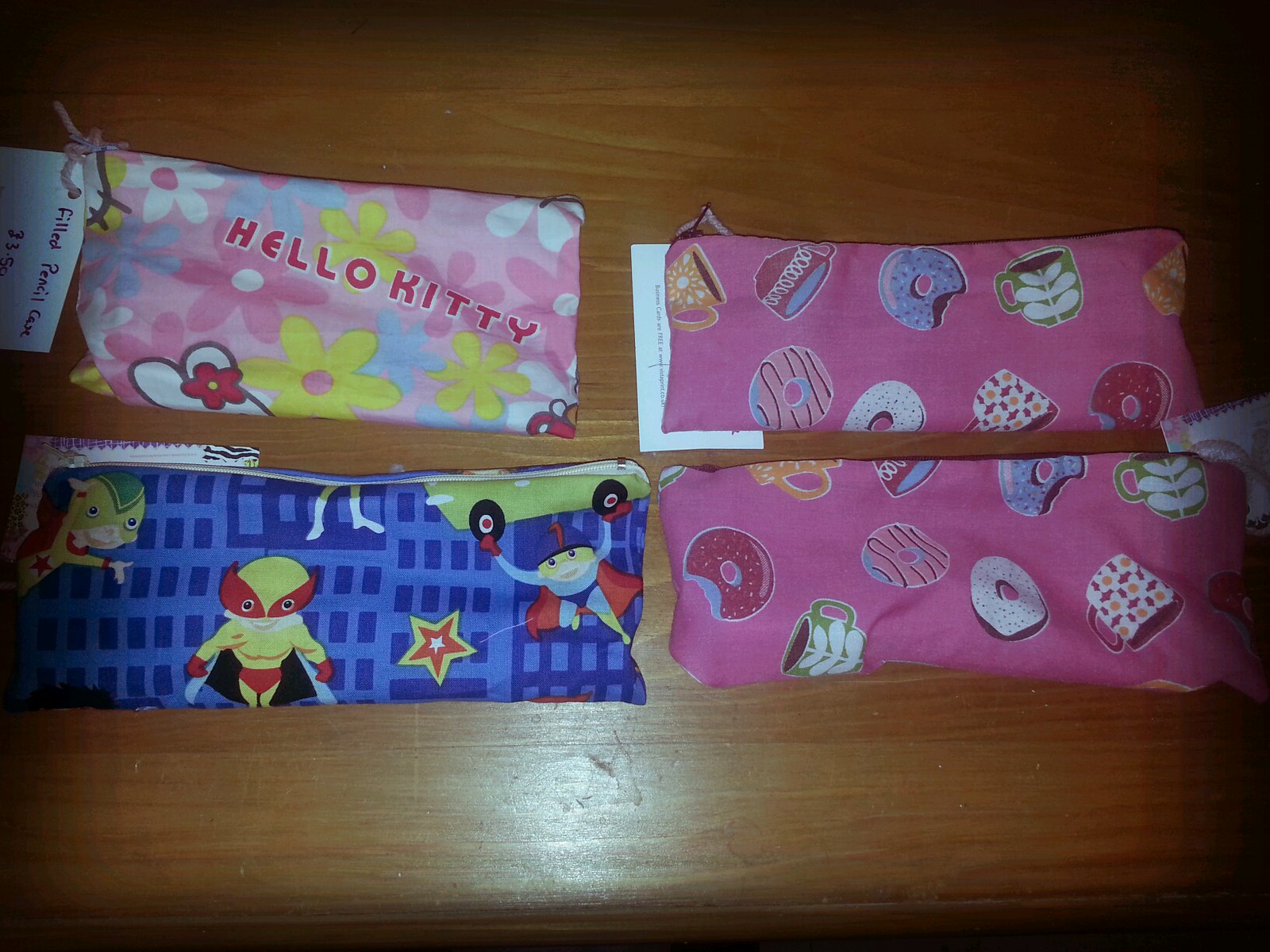This photograph depicts four distinct pencil cases arranged atop a wooden surface, which appears to be a dresser or table inside a house. The top left pencil case features a Hello Kitty design with multicolored flowers in yellow, blue, white, and pink, and displays the text "That Ticks" alongside "Hello Kitty." Both pencil cases to the right feature identical donut and coffee mug designs with variously colored donuts in blue, white, and pink. The bottom left pencil case showcases a cityscape with various masked superheroes, including one lifting a car above their head.